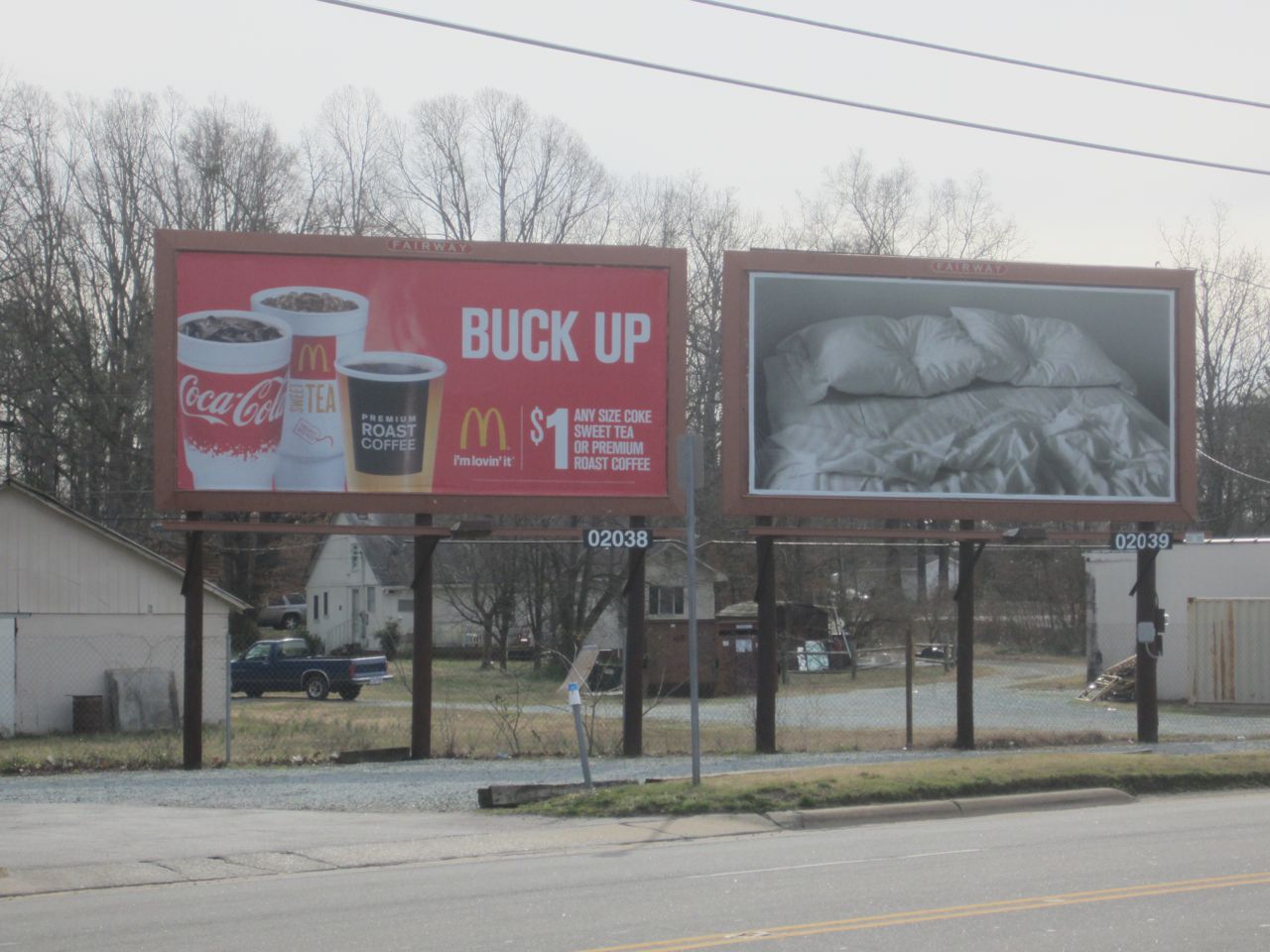The image depicts two billboards situated in an unkempt residential area. The picture, taken from across the street, captures a view of a nearby highway. 

The first billboard on the left is an advertisement for McDonald's. It prominently features the slogan "Buck Up" along with the iconic McDonald's logo and the phrase "I'm lovin' it." The ad promotes a deal offering any size Coke, sweet tea, or premium roast coffee for just one dollar. The billboard includes images of three drinks labeled as Coca-Cola, McDonald's Sweet Tea, and Premium Roast Coffee. Below this ad, the number "02038" is visible.

To the right, the second billboard, apparently owned by the same company, Fairway, shows a disheveled, unmade bed. The image hints at two people having just woken up, with noticeable impressions on the pillows and the blankets haphazardly wadded up. This billboard is marked with the number "02039."

In the background, a house can be seen alongside several dumpsters and scattered debris, contributing to the overall dilapidated appearance of the neighborhood.